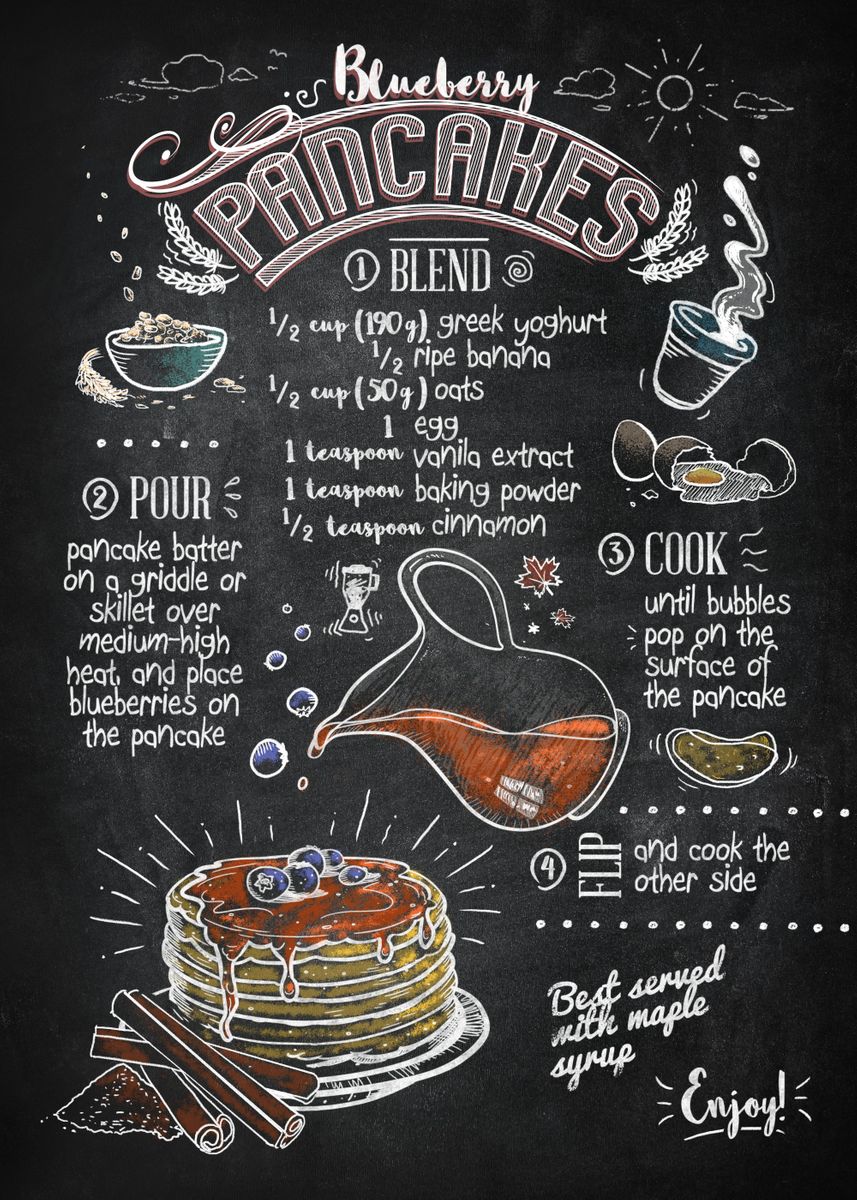The image resembles a professionally designed blackboard-style graphic, featuring a detailed recipe for blueberry pancakes. The background has a rich charcoal texture, not solid black, which gives it an authentic blackboard appearance. At the top, "BLUEBERRY" is written in white script, followed by "PANCAKES" in gray text underneath, both arched elegantly.

Central to the graphic are step-by-step cooking instructions and the necessary ingredients. "1. Blend" is accompanied by a list of ingredients: 1/2 cup (190 grams) Greek yogurt, 1/2 ripe banana, 1/2 cup (50 grams) oats, 1 egg, 1 teaspoon vanilla extract, 1 teaspoon baking powder, and 1/2 teaspoon cinnamon. 

"2. Pour" directs you to pour the pancake batter onto a griddle or skillet over medium-high heat and place blueberries on the batter. "3. Cook" instructs to cook until bubbles surface and pop. "4. Flip" advises flipping to cook the other side. Finally, the graphic suggests serving the pancakes with maple syrup, concluding with the word "Enjoy."

Scattered around the text are charming illustrations, including a sun and clouds, wheat shafts, oats, eggs, a hot cup of coffee, a salt shaker, and a brown pancake. Central to the visuals is a colorful stack of pancakes with blueberries, cinnamon sticks, and a clear pitcher pouring syrup. The lower middle emphasizes the syrup being poured onto the towering stack of pancakes, reinforcing the mouth-watering appeal of the recipe.